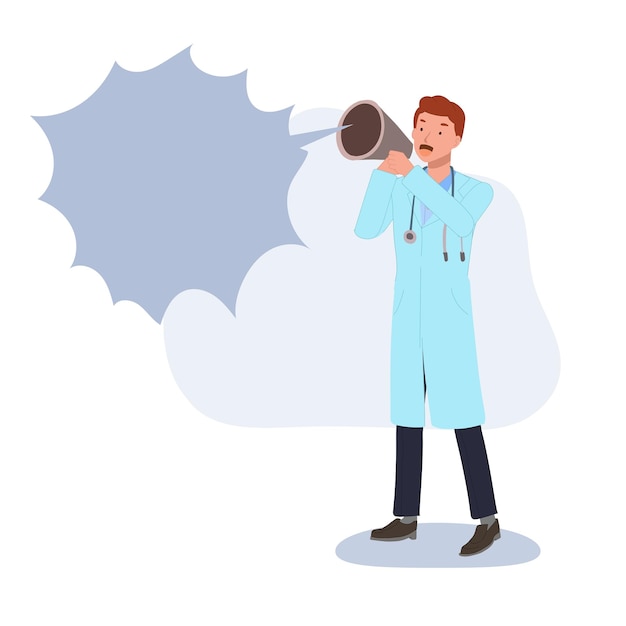This clip art style, simplistic digital animation features a white male doctor with curly red hair, appearing visibly angry as he shouts into a handheld gray megaphone. The doctor is dressed in a pale blue lab coat, with a slightly darker blue collared shirt beneath it, black pants, and brown dress shoes. A stethoscope is draped around his neck, reinforcing his medical profession. The doctor is standing on a gray disc against a completely white background, except for an oblong, misshapen light gray splotch behind him. Emerging from the megaphone is a jagged blue speech bubble, which is currently blank, inviting the viewer to add their own text. The doctor has both arms raised to his face as he holds the megaphone, facing to the left, with his mouth open in a shouting expression.